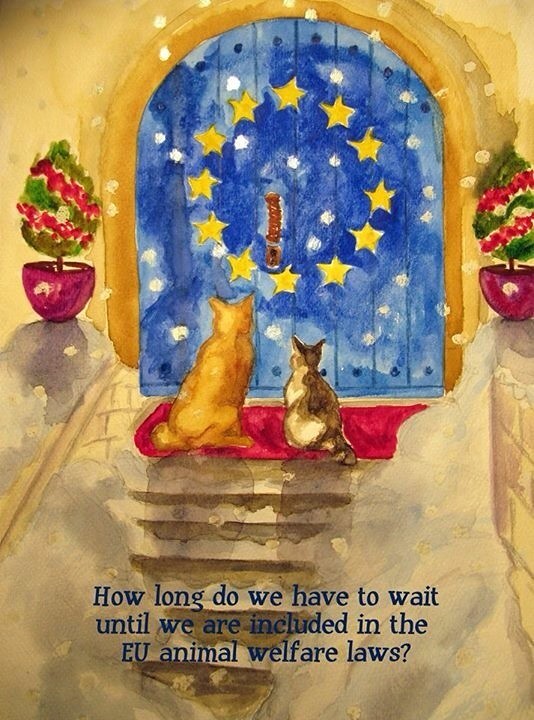In this detailed watercolor painting, a light brown dog and a black-and-white cat sit together at the top of snowy steps, gazing at a closed blue door adorned with white dots and yellow stars forming a circle around the handle. This whimsical door, framed by beige walls, is reminiscent of the EU flag. On either side of the entrance, potted plants with festive red ribbons add a touch of holiday cheer. A red floor mat lies at the threshold, emphasizing the sense of anticipation and hope embodied by the scene. The caption beneath the image poignantly asks, "How long do we have to wait until we are included in the EU animal welfare laws?", highlighting a call for improved and inclusive animal welfare regulations.